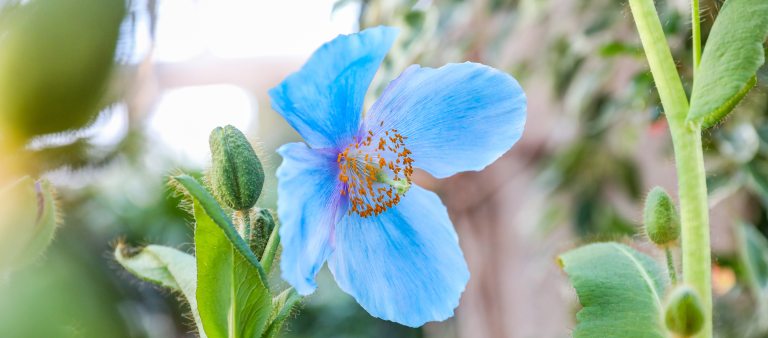This image is a close-up, horizontal photo capturing a vibrant blue flower in a natural setting, likely someone's backyard, during the daytime. The flower, almost neon in its brightness, features translucent petals with specks of purple and a striking orange pollen center. Surrounding the flower are at least four unopened flower buds. The background reveals a lot of greenery and a indistinct, blurred-out wall structure that appears light beige to reddish. The depth of field effect keeps the flower and accompanying green plants sharply in focus while rendering the background almost completely indistinguishable. The overall composition is dominated by the vibrant blue flower, devoid of any people, text, or other objects, making it the focal point of this serene nature scene.